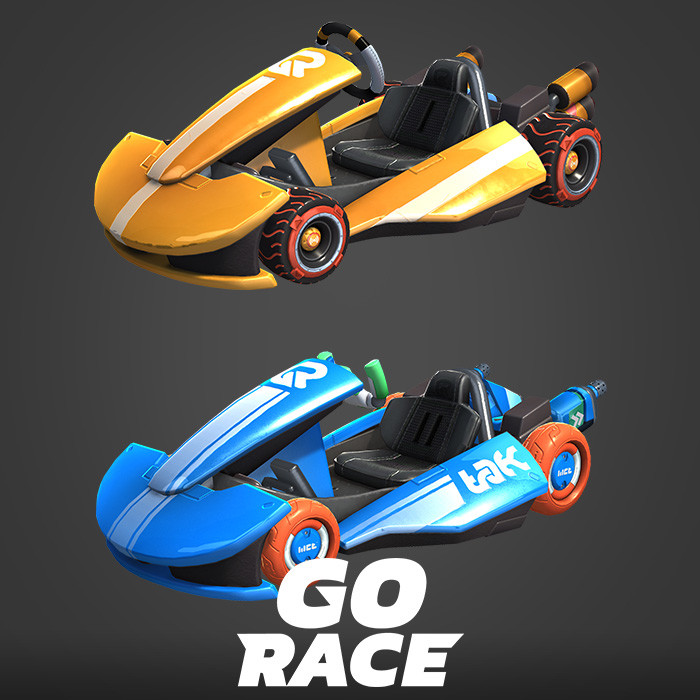This image is a detailed 3D rendering of two go-karts, resembling video game or concept art. Both karts appear to be nearly identical models, with differentiating features prominently highlighted. The background is gray, with a stylized "Go Race" text at the bottom in white.

The top go-kart is yellow with white racing stripes along its sides and center. Its tires are black with red trim, and it has a "GR" logo painted on the front. The steering wheel of this kart is circular, colored black and yellow, and the seat is entirely black. The tailpipes at the back are a combination of yellow and black.

The lower go-kart is blue with more complex white striping—one thicker stripe bordered by thinner ones, and two additional stripes down the front. This kart also features a "GR" logo on the front, along with a "TAK" marking on the side. Its tires are completely orange, differing in model from the top kart, and the steering wheel is a distinctive green and white half-circle shape. The steering wheel has green grips and serves as handlebars. The seat is black, and the tailpipes are blue. The overall design includes a low-to-the-ground frame and an exhaust system that extends from the back, designed like blue tailpipes.

Both go-karts have their unique elements while sharing a coherent aesthetic, making the image visually engaging and rich in detail.